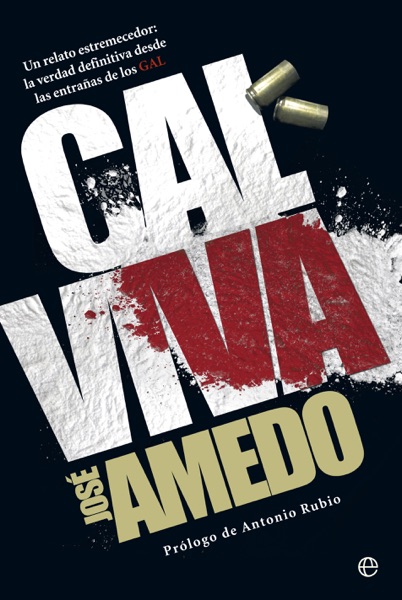The image appears to be a dramatic advertisement, likely for a book or a movie, presented as a computer graphic design. The central focus of the image is a text in Spanish, intricately arranged with various artistic elements. Against a solid black background, a tilted rectangular frame stretches diagonally from the lower left to the upper right. Within this frame, the dominant text is "VIVA," displayed in large, bold letters. The letters "I," "V," and "A" are notably stained red, resembling blood, while the rest of the text, in white, is textured to mimic broken-down cocaine. Flanking the text are two bullet casings positioned in the upper right corner, adding a sense of urgency and drama.

Above this main text, in small white letters, the phrase "Un reto estremecedor la verdad definitiva desde las entrañas de los GAL" is written, with "GAL" highlighted in red. At the bottom, the name "José Amedo" appears in a goldish, cream color, followed by "Prólogo de Antonio Rubio" in white. Completing the design, a circular logo is placed in the bottom right corner, featuring an interlacing line pattern, underscoring the gripping and intense nature of the advertisement.